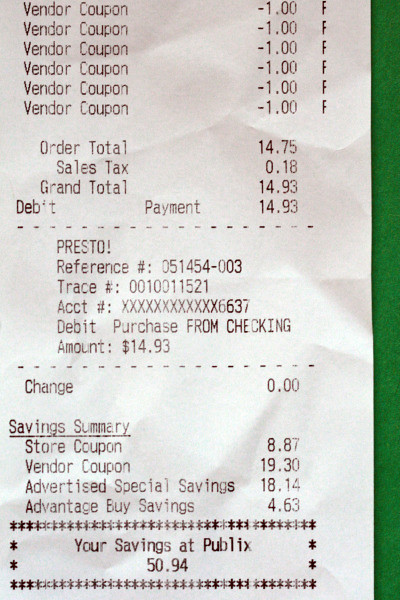The image shows a white receipt with black text against a green background. At the top left, the phrase "Vendor Coupon" is repeated six times, with each line showing a "-1 F" on the right. Below these, the receipt details: Order Total: $14.75, Sales Tax: $0.18, Grand Total: $14.93, and Debit Payment: $14.93, followed by a dashed line. Continuing, it states "PRESTO!" with a reference number (051454-003) and a trace number (0010011521). Details include an account with a debit purchase from checking amounting to $14.93, and change given, which is $0. In the Savings Summary, it lists Store Coupons: $8.87, Vendor Coupons: $19.93, Special Savings: $18.14, and Advantage Buy Savings: $4.63. The bottom of the receipt, framed in a box made of stars, declares "Your Savings at Publix: $50.94."